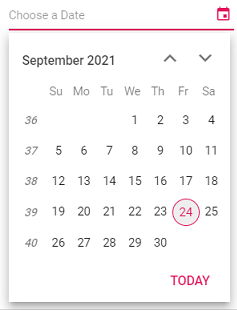The image features a light purple background with the heading "Choose a Date" at the top. In the top-right corner, there is a small light purple calendar icon with a purple square. A purple line runs horizontally across the top of the image. Below this line, the text "September 2021" is displayed, accompanied by an up arrow and a down arrow for navigating through months. The days of the week are listed from Sunday to Saturday. 

The calendar itself details the days from the 1st to the 30th. On the left margin, starting from the first row of the calendar, the numbers 36 through 40 are listed. Notably, the 24th of September is highlighted with a purple circle; the number 24 is also purple, and the circle has a light purple fill. The word "Today" is written in a light purplish-pink color. The entire calendar is set against a light purple background, adding a cohesive and soft aesthetic to the overall design.